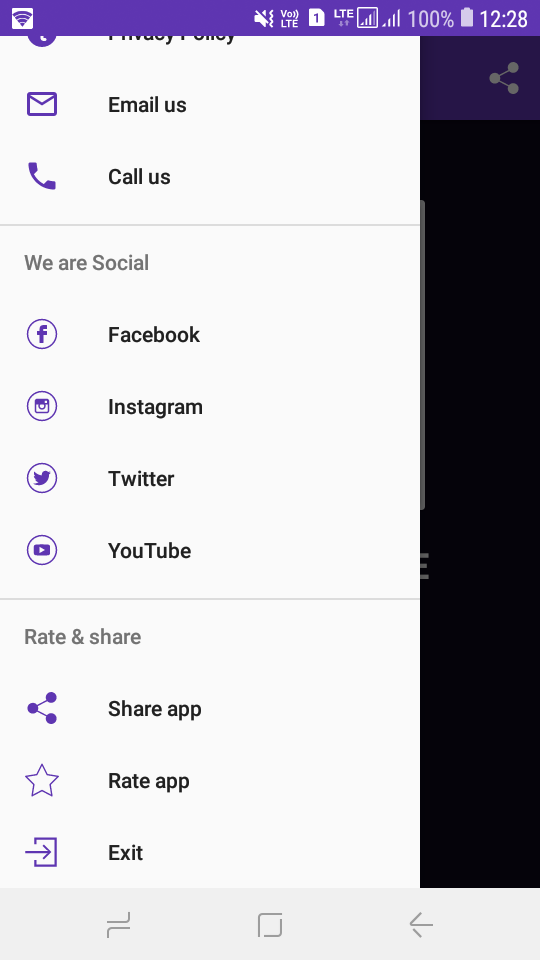Screenshot of a smartphone displaying a section of a web page with various contact and social media options, each represented by purple icons. The status bar shows the phone is on LTE with 100% battery and sound turned off. At the top of the list, the first option is unreadable, followed by "Email Us" with an envelope icon, and "Call Us" with a phone icon, both in purple. Further down, there are social media links under "We Are Social," each displayed in purple circles: Facebook (F), Instagram (camera), Twitter (bird, now X), and YouTube (play button). Additionally, options to "Rate and Share" the app are available, including "Share App" and "Rate App" with a star and "Exit" symbolized by an arrow through a door. The background is predominantly white with black text, bordered by a black bar on one side.